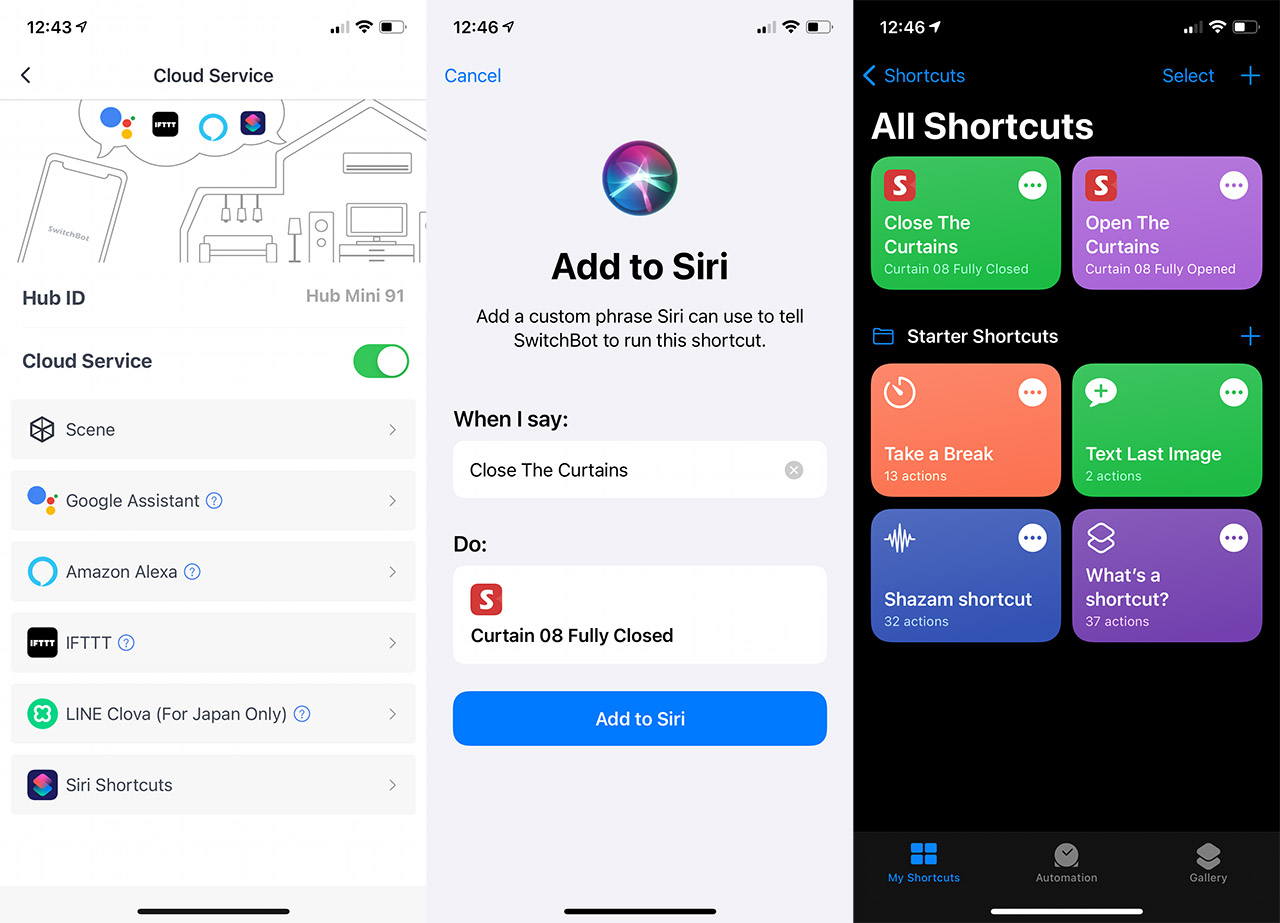This image displays three cell phone screens aligned horizontally, each showcasing distinct interfaces and background colors. 

The first screen, with a white background, displays the current time as 12:43 and shows a battery level at approximately 50%. At the top, the header reads "Cloud Service." Just below, there is a graphic of a house and a phone, symbolizing communication. Underneath the graphic, the text reads "Hub ID" in black, followed by "Hub Mini 91" in gray. Further down, "Cloud Service" is written again in black lettering, next to a switch that's toggled to the "on" position, indicated by a white circle on the right side with a green background to the left. Six options under "Cloud Services" are listed sequentially: Scene, Google Assistant, Amazon Alexa, IFTTT, Line Clova (for Japan only), and Siri Shortcuts.

The second screen, featuring a gray background, shows the time as 12:46 and approximately 33% battery life. The top left corner of the screen has a blue "Cancel" button. Beneath it, a circle with a wavy light design is central, above the large text "Add to Siri" in black. In smaller text, "Add a custom phrase Siri can use to tell SwitchBot to run this shortcut" is explained. Following the text "When I say," a white search panel contains the phrase "close the curtains." Below this, the text "Do" leads to another white field, which displays a red square with a white 'S' logo, followed by "curtain 08 fully closed" in black text. Two buttons dominate the lower part of the screen: a red button at the top, followed by a blue "Add to Siri" button in white text.

The third screen, with a black background, also shows the time as 12:46 and a battery level at about 50%. Positioned at the screen's top, blue text reads "Shortcuts" on the left and "Select" on the right. The text "All Shortcuts" is displayed prominently in white just below. Two squares occupy the central part: a green one labeled "Close the curtains" and a purple one labeled "Open the curtains," each featuring a red square with a white 'S' logo at their top left corners. The lower part of the screen is headed "Starter Shortcuts" in white against the black background, with four squares displayed in two rows and two columns. The top left square is orange and titled "Take a break," the top right square is green with "Text last image," the bottom left square is blue with "Shazam shortcut," and the bottom right square is purple with "What's a shortcut." At the very bottom, typical cell phone icons are lined up.

This detailed layout encapsulates various steps to setting up and using smart home shortcuts via voice commands through different apps and services displayed on the three phone screens.